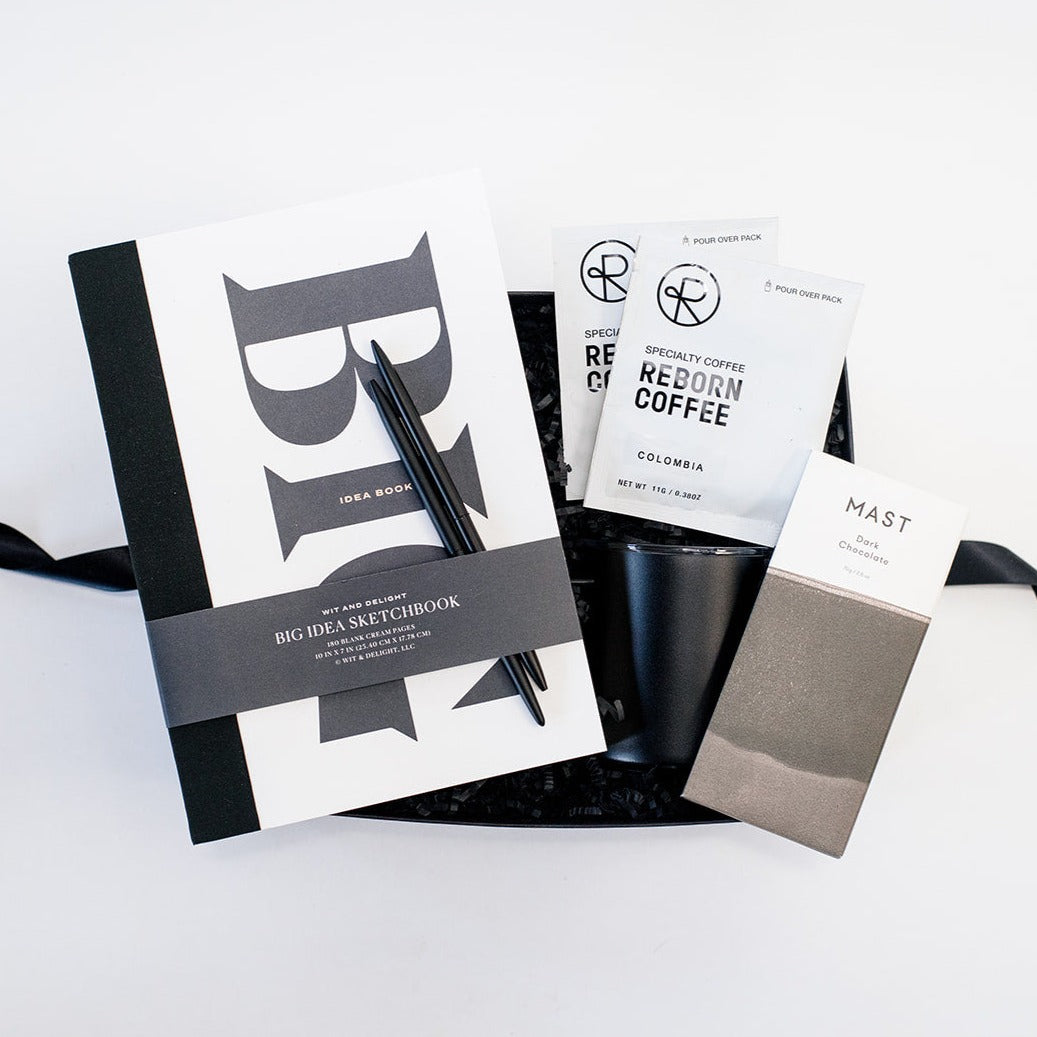The image is a square-shaped collection of assorted items, all presented on a pristine white background. On the left side, there is a black-and-white sketchbook with a large vertical inscription of the word "BIG" in dark gray letters, and the phrase "IDEA BOOK" in smaller text within the 'I'. Around the sketchbook, a ribbon is wrapped, displaying the text "BIG IDEA SKETCHBOOK," with a couple of pencils tucked neatly between the ribbon and the book. Next to the sketchbook, there are two white packages with black lettering that read "Specialty Coffee" and "Reborn Coffee, Columbia." Positioned below these is a sleek black coffee cup. To the right of these items, a white and gray packaged item marked "MASKED Dark Chocolate" is visible, suggesting it is a chocolate bar. All these items appear to be arranged within or in front of an open gift box with black ribbon and decorative confetti paper peeking out from behind, enhancing the curated and thoughtful nature of the collection.